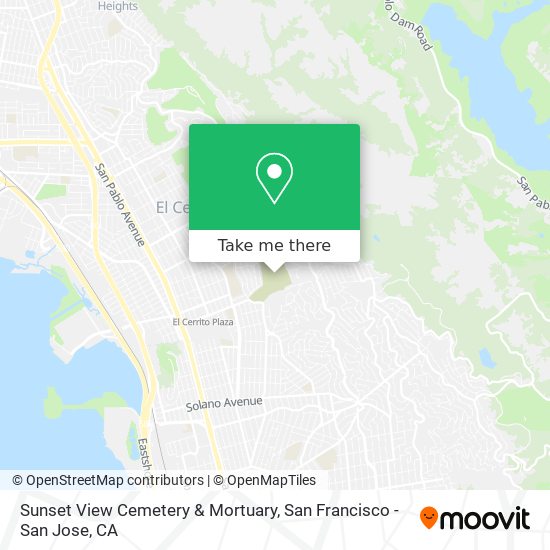The image is a colorful, square-format screenshot from the Moveit app, displaying a detailed map that features a variety of landmarks and labels. Prominently featured in the bottom right corner, the Moveit logo comprises black text reading "MOOVIT" alongside an orange, upside-down teardrop-shaped smiley face. At the bottom of the app, credits are given to OpenStreetMap Contributors and OpenMapTiles, as well as referencing the Sunset View Cemetery and Mortuary, San Francisco - San Jose, California.

In the central section of the map, there is a notable green square marked with a white, upside-down teardrop symbol indicating a point of interest. Directly below this symbol, the green square transitions into a white horizontal band containing the black text "Take Me There." Surrounding this focal point, the map is rendered in light blue, light green, cream, and gray, with detailed white rows running diagonally from the top left to the bottom right. 

Key landmarks include a pool area or body of water situated at the bottom left and a narrow water body located at the top right. Prominent geographical labels on the map also include San Pablo Avenue and El Cerrito Plaza. The style of the map blends color illustration with text and graphic design elements, effectively guiding the user to the selected location.